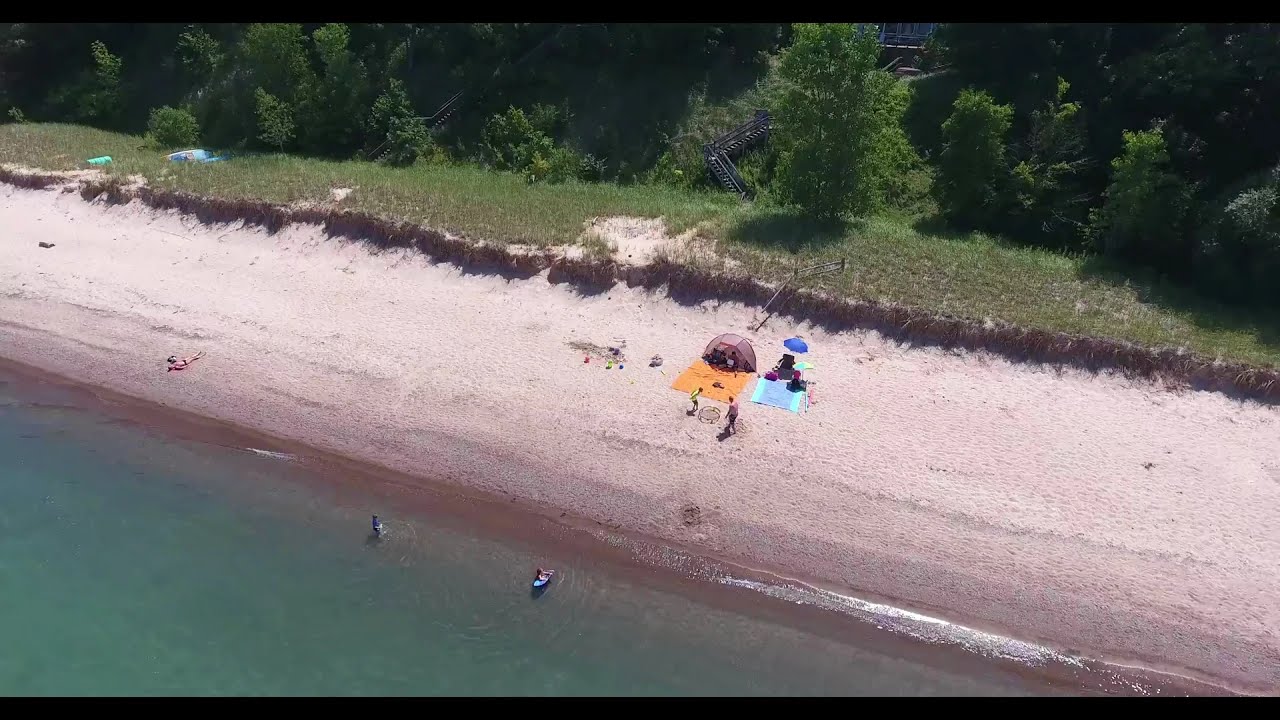This aerial photograph captures a beach scene taken from approximately 50 feet above with the camera angled down at about 45 degrees, providing a detailed view of the landscape. The beach lies at the edge of a murky green body of water, shaping a right triangle in the lower left of the image. The water meets the beach with a hint of white foam and transitions from darker clay at the water’s edge to light, almost white sand. 

On the beach, two sunbathers occupy a spot with an orange towel and a blue towel. A black Speedo-clad man lies to the left, while a gold-yellow beach tent set up over one towel shelters a person. The adjacent blue towel is accompanied by a beach chair and a blue umbrella. Nearby, two additional people are engaged in the water, one with arms extended over a boogie board and the other, a child, standing up. In front of the blankets, two individuals stand in a small circle on the sand.

The beach area is bordered by a grassy embankment which transitions into a dense arrangement of trees stretching around the beach edge. Behind the beach, partially concealed by a large tree, is a wooden staircase leading up to a house, nestled amongst the foliage. The entire scene is bathed in daylight, highlighting the varied textures and colors of the beach and its surroundings.